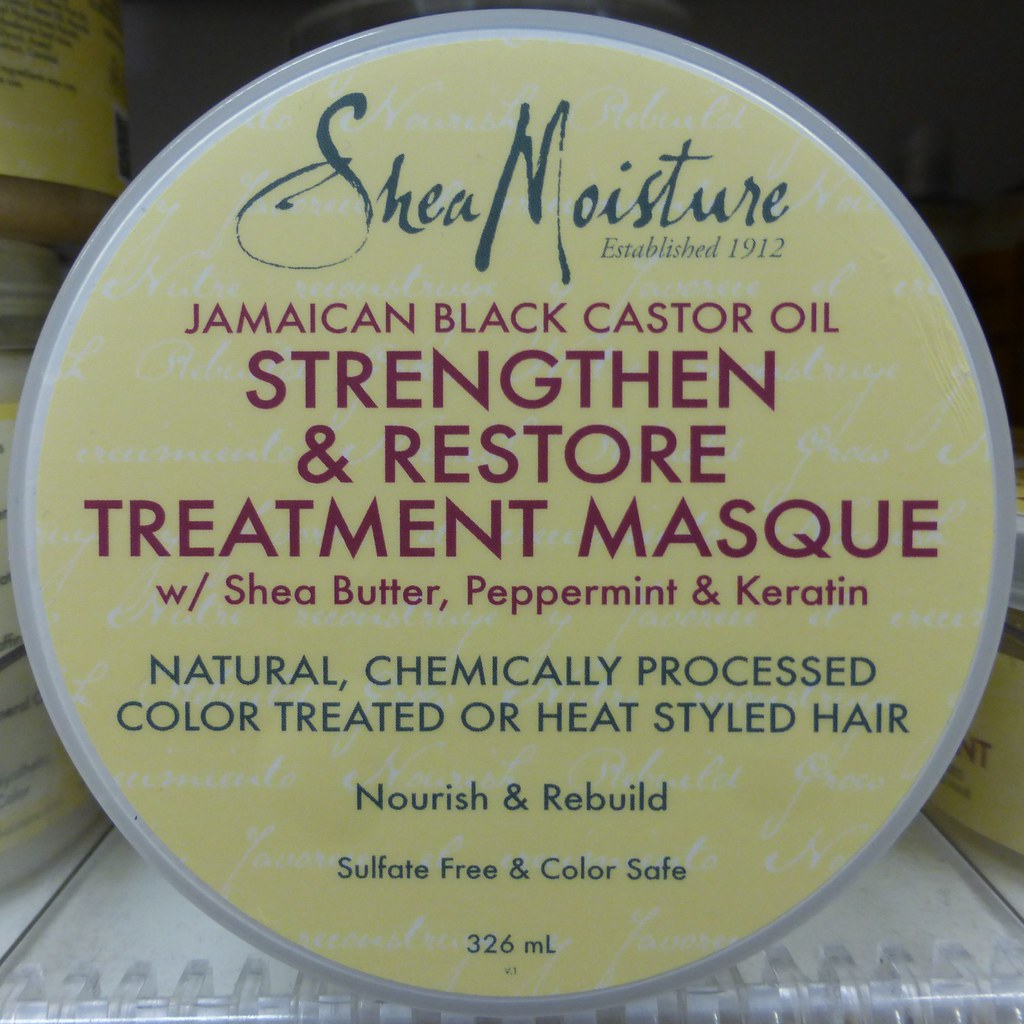The image features a zoomed-in view of a circular plastic lid, likely a cap or screw-on lid from a product jar. The background of the lid is a very pale yellow, almost pastel in shade. At the top of the lid, the logo "Shea Moisture" is displayed in a green, handwritten cursive text, with "Established 1912" written in small black text underneath. The main body of the text is in different colors: "Jamaican Black Castor Oil Strengthen and Restore Treatment Mask" is prominently written in maroon, with "Mask" spelled "M-A-S-Q-U-E." Below this, in smaller maroon text, it reads "With Shea Butter, Peppermint, and Keratin." Towards the bottom, dark green text states "Natural, Chemically Processed, Color Treated, or Heat Styled Hair," and further below, it says "Nourish and Rebuild, Sulfate-Free and Color Safe, 326 milliliters." The lid is situated on what appears to be a plastic shelf, with several similar products visible in the background.